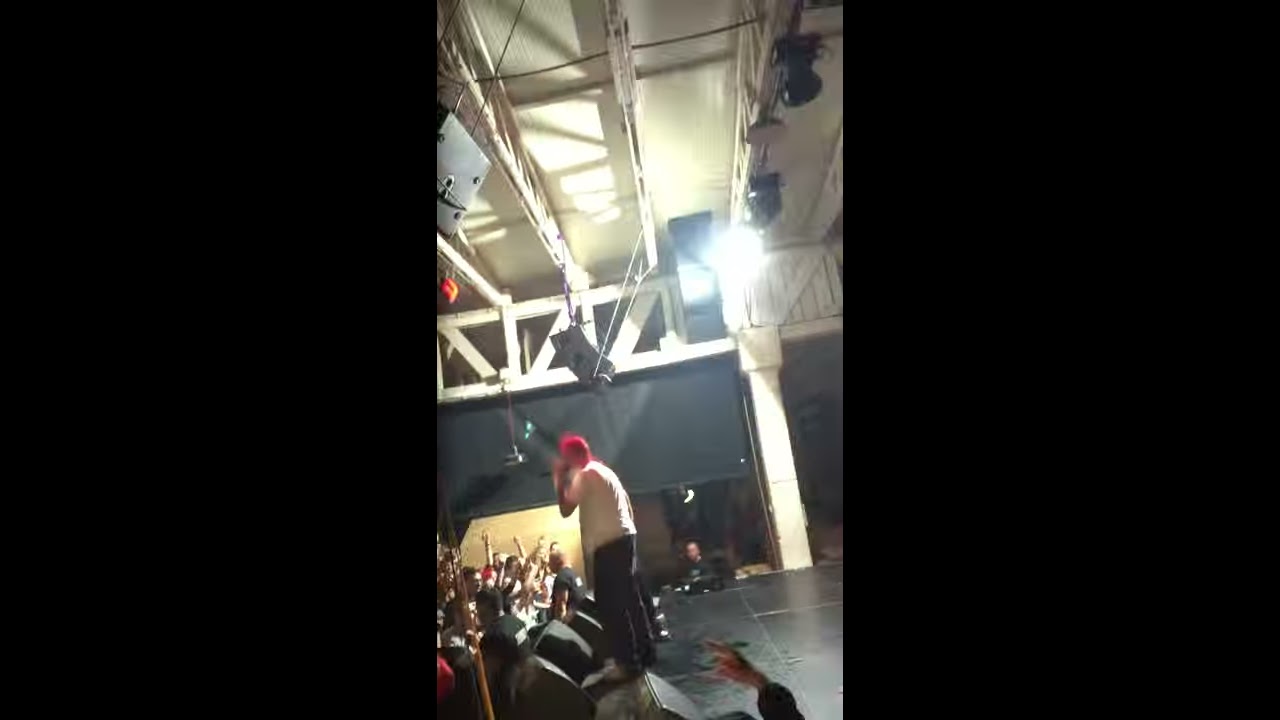The photograph depicts a nighttime scene inside a concert hall, with a man wearing a white shirt, dark pants, and a red baseball cap standing on a black, shiny stage. He is holding a microphone close to his mouth, singing to an enthusiastic crowd. The lighting is provided by an overhead light hanging from white rafters that are supported by a pillar. Above the man, there is a white catwalk and possibly a large black speaker suspended from the ceiling. The audience in front of the stage is animated, with many members waving their hands, suggesting they are dancing or celebrating. The background features a brown wooden wall, and the sides of the image are framed by large black rectangles, which dominate more than half of the photo and add a dramatic, focused effect on the central subject. There is no text in the photograph.